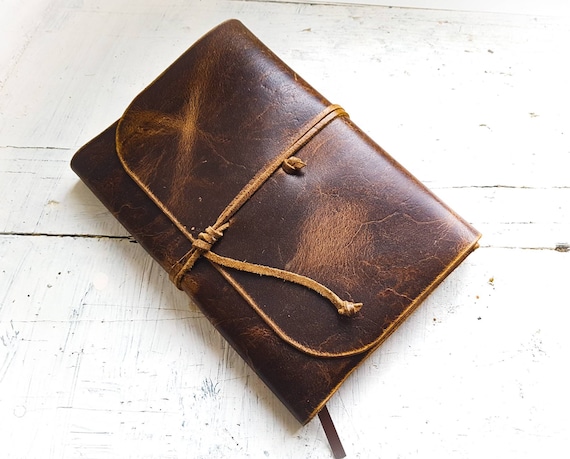This detailed photograph features a worn, brown leather clutch purse, reminiscent of cowhide, resting on a clean, white surface that could be a table or a floor. The clutch exhibits a two-tone effect with lighter beige hues mixed into its darker brown leather, suggesting a natural patina from use. The purse, designed like a small envelope clutch, is secured by a vertical leather tie rope that hangs off to the right. The bright lighting in the image highlights the texture and worn spots on the leather, indicating it has seen some use. The minimalist white background enhances the focus on the purse, suggesting it might be photographed for a sales listing, possibly on a website like eBay.